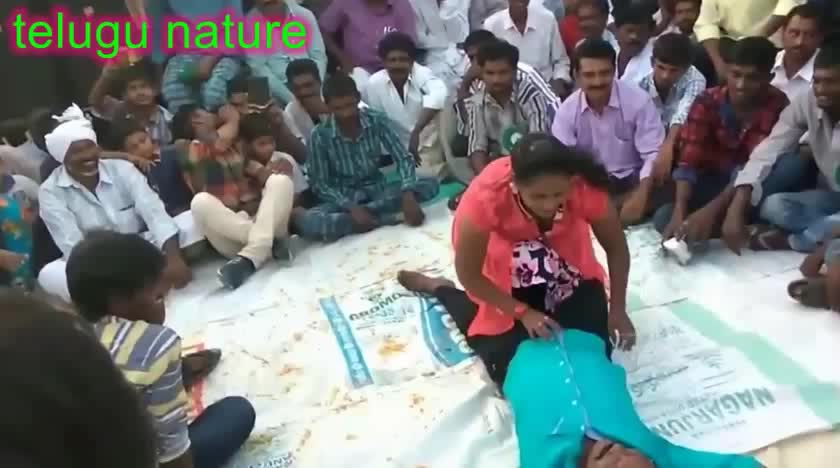In this detailed landscape photograph, a group of Indian or Pakistani men and boys with dark complexions and black hair sit on the floor in a semicircle, three to four rows deep, with varied, colorful clothing and expressions ranging from amusement to indifference. They are surrounding an intriguing scene: a man in a turquoise long-sleeve shirt and black pants lies on a large white banner or advertisement adorned with unreadable blue text. Atop him, a woman wearing a short-sleeve pink blouse with white and pink floral patterns squats, possibly performing a massage or a balancing act. Her dark, fluffy hair obscures part of her face as she focuses downward. The setting is further contextualized by embossed text in light green with a pink shadow in the upper left corner, reading "Telugu nature," indicating a local or cultural significance. Additionally, one man wearing a distinct white turban and white attire stands out on the left side of the gathering, adding a unique visual element to the diverse congregation.